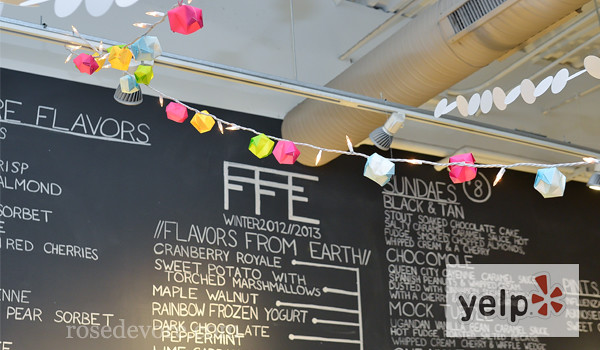The image depicts a black chalkboard menu, located inside a restaurant, featuring white chalk text. The board prominently displays "FFE, Winter 2012-2013, Flavors from Earth" in the middle, and lists various flavors such as cranberry royale, sweet potato with torched marshmallows, maple walnut, rainbow frozen yogurt, dark chocolate, and peppermint. Additionally, sundae options including Black and Tan, Chocomole, and Mock Turtle are listed on the right side. The bottom right corner of the chalkboard showcases a Yelp logo with a white box, black text, and a red logo, seemingly photoshopped onto the image. The restaurant's ceiling is adorned with several decorations, including what appear to be cardboard boxes and strings of multicolored lights in red, yellow, green, and blue.